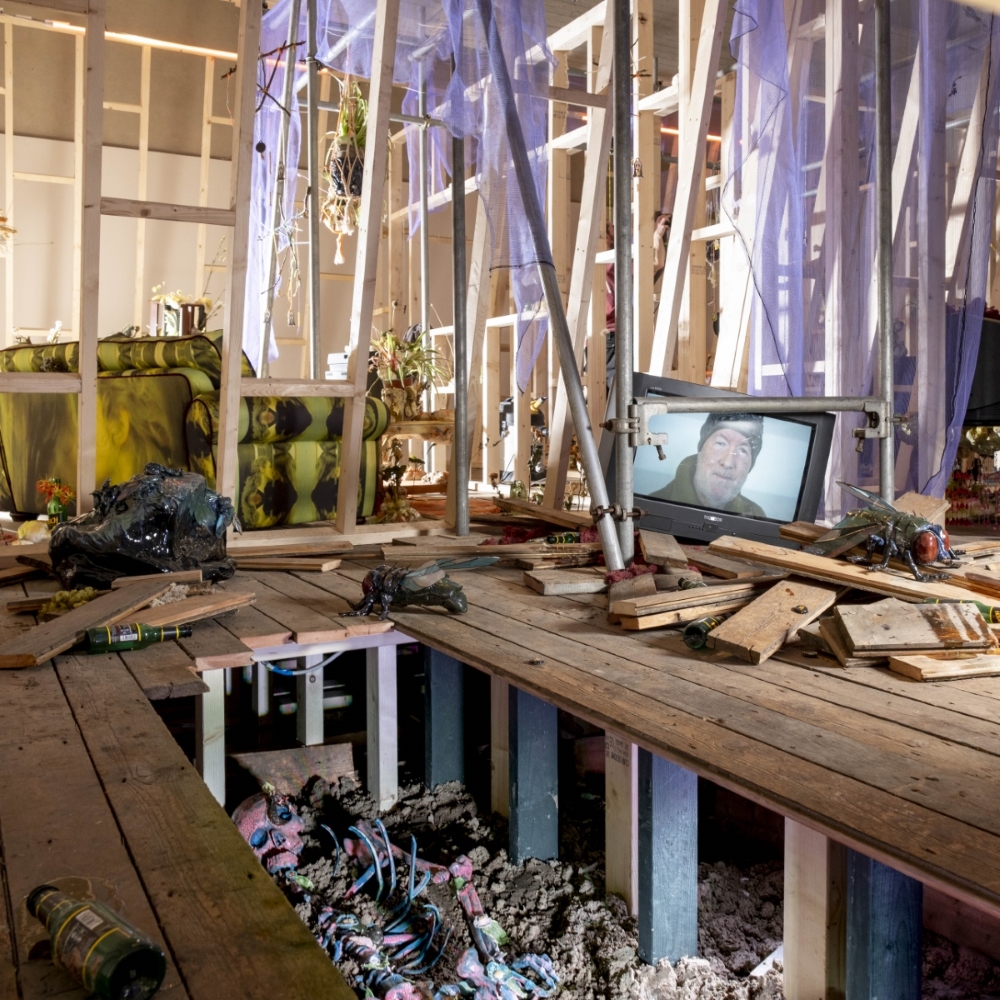The image depicts a chaotic construction site, likely the interior of a home on the ground or basement level. The area is filled with wooden 2x4s and other lumber, both stacked and scattered around, suggesting an incomplete structure with exposed framing and beams. Sunlight streams in from above, illuminating the scene. The floorboards have been removed, revealing dirt and debris underneath, including an unusual blue and purple skeleton—possibly a prop. Amongst the disorder are various items such as metal poles, beer bottles, and random junk. Notably, there’s a small digital screen or TV showing the face of a man in a black hat, oddly juxtaposed with a giant statue or figure of a fly, adding a surreal element to the construction chaos.